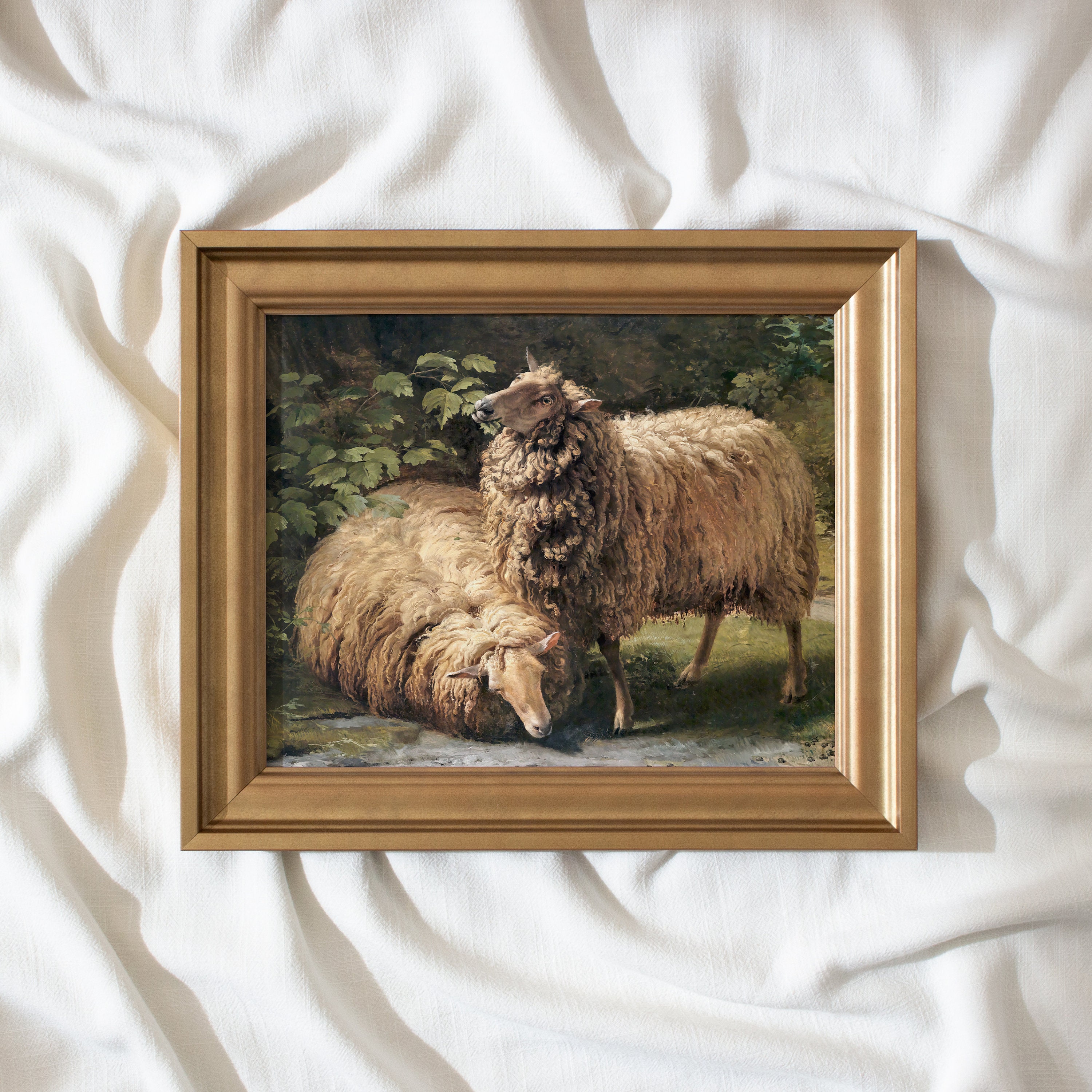This image features a professionally framed drawing or oil painting of two sheep set against a crumpled white linen fabric backdrop to add texture. The soft gold, matte frame enhances the artwork, which portrays an idealized natural scene. Both sheep are depicted in golden hues rather than brown, with the one on the right standing and gazing into the distance, while the other lies down, appearing to look at the ground. The sheep shown have thick, textured wool with deep shadows. The setting includes patches of green grass and gray stone, giving a natural yet slightly stylized impression. On the left side of the image, bushes, leaves, and perhaps a tree contribute to a background suggestive of foliage and nature.